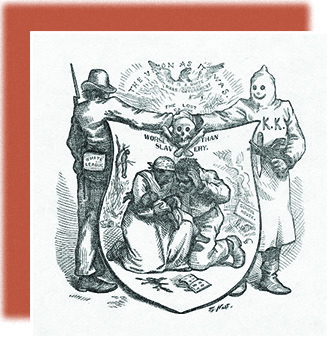This black and white drawing, possibly an etching or a penciled political cartoon from the Jim Crow or post-abolitionist era, serves as a stark depiction of historical racism. Central to the image is a shield-like crest containing a sorrowful scene of an African-American family: a man and a woman, both kneeling and seemingly shielding their anguished faces while holding a baby, suggesting desperation and fear. Above them looms a stark and grisly skull, symbolizing death or oppression.

On either side of this crest, two figures reach towards each other, clasping hands over the skull. To the left stands a man in coveralls and a hat, reminiscent of a farmer or a slave bounty hunter, brandishing a rifle with a bayonet. Opposite him is a sinister figure in a white robe and hood, emblazoned with "KKK," indicative of a Ku Klux Klan member. They depict a grim alliance, their handshake over the emblem of death reinforcing their shared animosity.

In the background, partially obscured text includes the phrases "the … as it was," hinting at a nostalgic or reactionary sentiment. Additionally, there is a haunting image of a figure lynched and hanging from a tree, underlining the violence of the era. Supplementing the main illustration is an orange square positioned behind it, akin to a drop shadow. Completing the scene, a book and a spilled ink bottle lie at the enslaved family's feet, adding to the sense of despair and abandonment.

The image is surrounded by brown borders along the top and left sides, emphasizing the historical context within which these atrocities were recorded and remembered. The artwork might also include the artist’s signature, grounding this depiction in a specific historical moment and perspective.